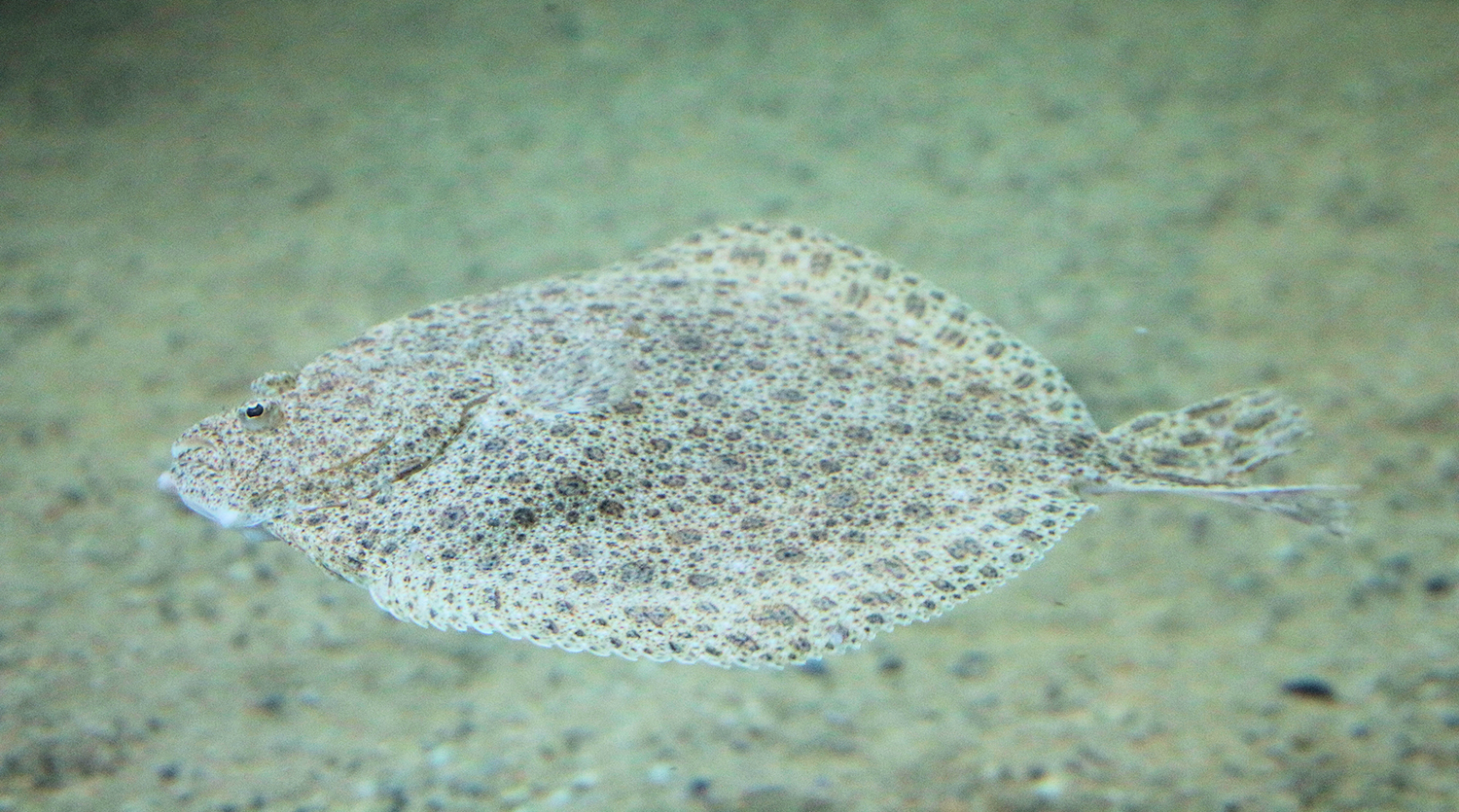This is a clear and close-up photograph of a very flat fish, most likely a flounder, laying on the sandy bottom of the water. The background is predominantly sandy, featuring muted tan colors with specks of white and black. The fish itself appears camouflaged, its body covered in scattered spots and speckles of gray, brown, and black circles against an off-white base color. The fish is shaped somewhat like a pancake, with a broader top section tapering down to a narrow tail, which is also speckled and appears triangular or heart-shaped. You can distinctly see its black eye on the left side of the photograph, along with what looks like its mouth. The body of the fish is thin but wide, blending seamlessly with the sandy environment around it.